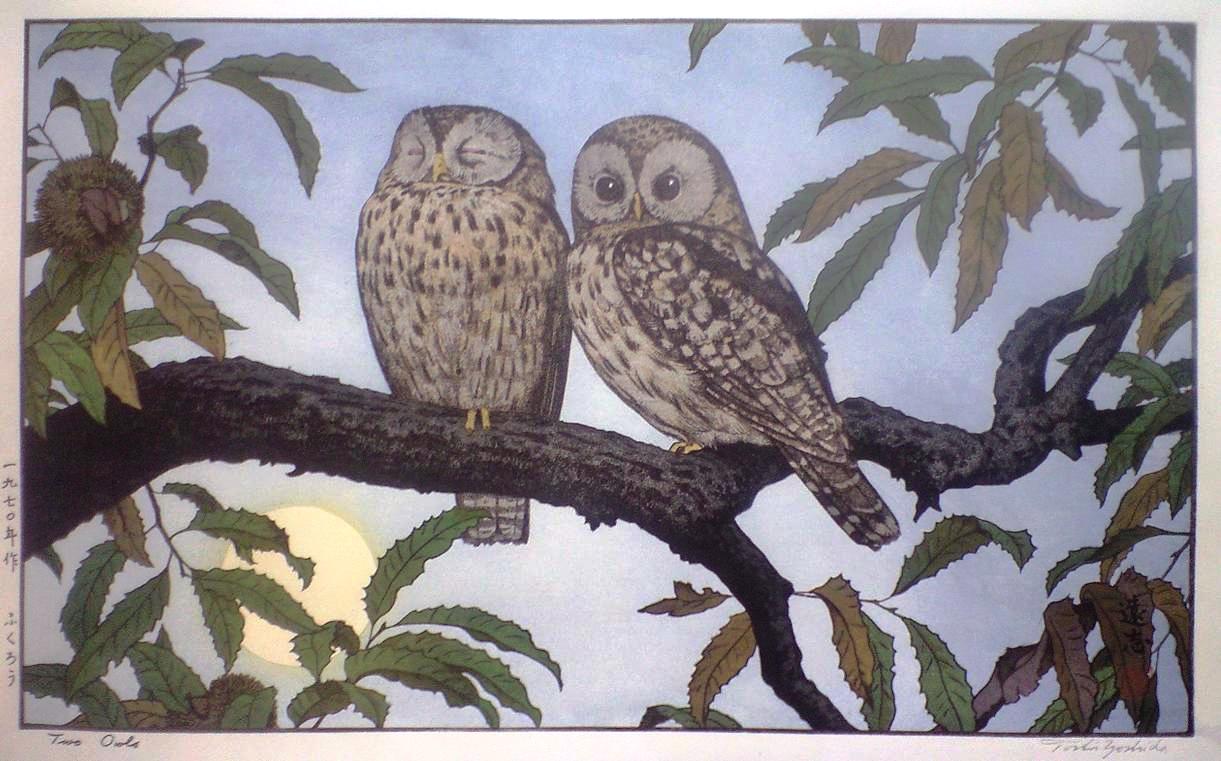This detailed illustration features two nearly identical owls perched on a large, predominantly brown tree branch. The branch, adorned with a mixture of green, tan, grey, and yellow leaves, is set against a light blue sky with a glowing yellow moon in the background. The owl on the left, with its eyes closed, clutches the branch with a single yellow claw. It is mostly tan with grey spots and has a yellow beak. The owl on the right, also mostly tan with grey spots, has more of its wing visible, displaying a dark grey line. This owl gazes outward with open eyes. Both owls share similar features, including yellow beaks and feet, adding to the intricate texture and depth of the artwork.